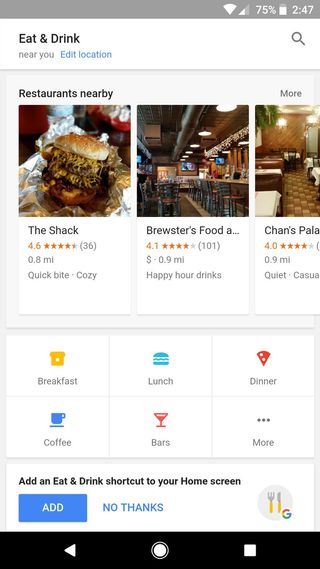A screenshot on an Android device showing a web browser search for restaurants, likely using Google. The interface is within a section labeled "Eat and Drink – Near You," which features a button to edit the location. Three highlighted restaurants are visible, each with an image and name: 

1. "The Shack," showcasing a mouth-watering, high-calorie burger with juicy meat and onion rings. 
2. "Brewster's Food," which presents itself as a bar-style eatery.
3. "Chan's Palace," a sophisticated Asian restaurant.

The interface suggests that additional restaurant options can be revealed by scrolling to the right. At the bottom of the screen, there is a prompt to "Add an Eat and Drink shortcut to your home screen," with "Add" and "No Thanks" buttons available. A subtly placed Google logo is seen at the bottom right corner. Additional navigation buttons labeled Breakfast, Lunch, and Dinner allow further exploration of meal-specific options.